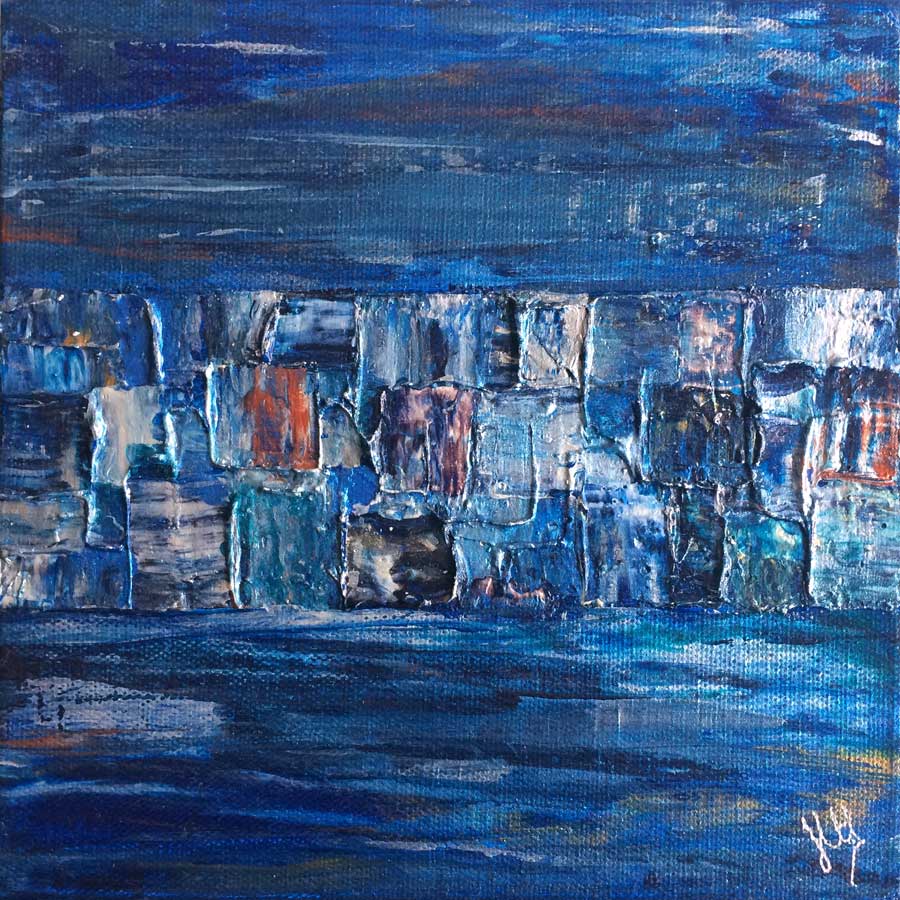This abstract painting, likely created with oil or acrylic paints on canvas, features a predominantly blue color palette with shades ranging from dark blue to turquoise, accented with hints of white, reddish, pink, and purple. The composition is divided into three horizontal sections. The top and bottom sections consist of horizontal streaks and swishes of color, creating a flat and uniform appearance. In contrast, the middle section is more textured and dynamic, characterized by raised, thick paint applied with a motion that forms almost perfect square shapes. These squares are filled with varied, multicolored patches, adding depth and complexity to the center of the artwork. The overall mood of the painting is somber, conveyed through the cool, blue tones and the angular, geometric forms. The artist's initials, painted in white cursive, are located in the bottom right-hand corner of the piece, providing a subtle signature to this textural and emotive abstract work.